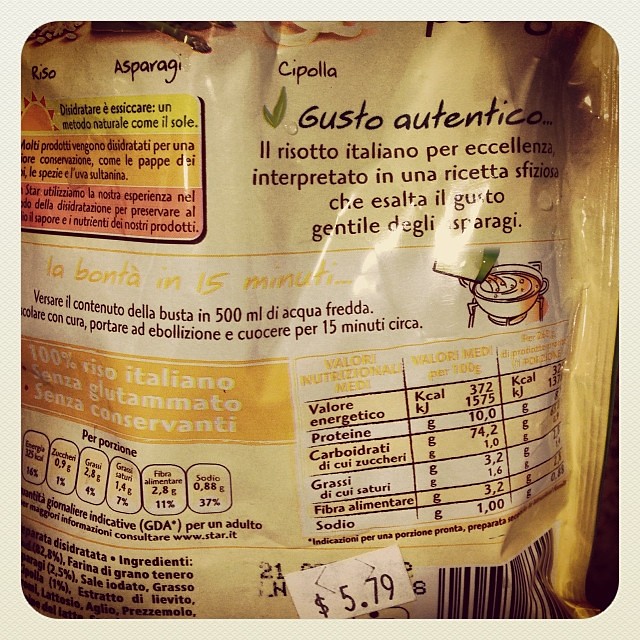**Detailed Caption:**

This is a close-up color photograph featuring a square image with a distinctive white border. The outer corners of the bordered frame are square, but the inner edges are rounded, giving a soft touch to the overall appearance. The image captures the back of a food package, likely a resealable plastic bag, printed with vibrant text and graphics.

The package appears to be an Italian product, as indicated by the text "Gusto autentico il risotto italiano per eccellenza interpretato in una ricetta spiziosa," suggesting an authentic and exquisite Italian risotto recipe. However, upon closer inspection of the ingredients listed as "farina, grano tenero," it becomes evident that the product is made from wheat flour, implying it might be a type of pasta rather than rice.

The top of the package is labeled with "Riso Asparagi Cipolla," which translates to "Rice, Asparagus, Onion," indicating either the flavor profile of the product or other varieties offered by the brand. Below, there is an eye-catching text box featuring an orange sun icon with radiant red rays, and several colorful bars displaying important nutritional information and product highlights.

There is a white price sticker marked at $5.79, oddly placed over the best by date, making it partially obscured. On the bottom right corner, a UPC or barcode is visible, accompanied by detailed nutritional values listed in both kilocalories (kcals) and kilojoules (kJ). The nutritional breakdown includes proteins, carbohydrates (noted as "carboidrati" and "decuisucari" for added sugars), fats ("grassi" and "decuisaturi" for saturated fats), dietary fiber ("fibre alimentari"), and sodium ("sodio"). 

Overall, this photograph intricately showcases the packaging details of what appears to be a premium Italian food product with a focus on its nutritional content and authentic flavor profile.